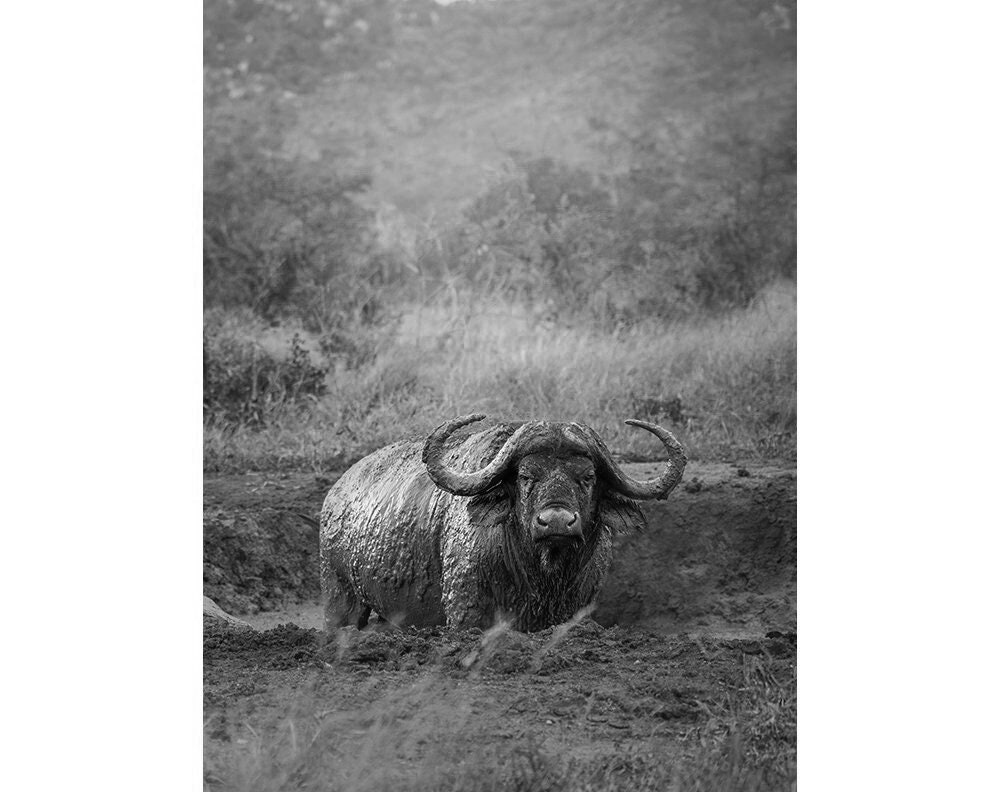The image depicts a surreal, computer-generated water buffalo standing in a muddy crater within a marshy area. Rendered entirely in shades of gray, the buffalo's features are unsettlingly human-like, including a smiling mouth, eyes, and nose seamlessly blended with its natural facial features. The water buffalo, covered in dripping mud, is looking directly at the viewer with curved horns reminiscent of a handlebar mustache. In the background, the muddy scene is framed by indistinct trees and tall, dried grass, which add to the eerie and fantastical nature of the artwork. The details merge into a striking, monochromatic portrayal of a half-human, half-buffalo creature amidst its peculiar, marshland habitat.